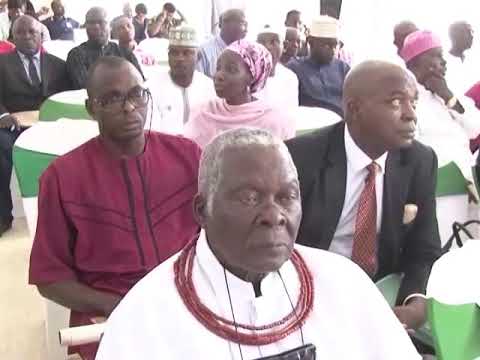The photograph portrays a gathering of predominantly African or African American men and women seated in a large hall, suggesting a conference or seminar setting. The attendees are seated on green and white chairs with no tables visible, contrary to the initial perception. The atmosphere is serious and stoic, with no visible smiles among the participants. The men are predominantly dressed in black business suits, while others are adorned in traditional African attire, such as white daishiki-like garments and rimless caps. A notable woman in the center wears a pink and black head wrap and a pink shawl. Another man, positioned towards the front, dons a red linen short sleeve shirt. The attire and gathering suggest a formal event, possibly religious or cultural, with participants facing various directions, indicating the event might not have started yet.